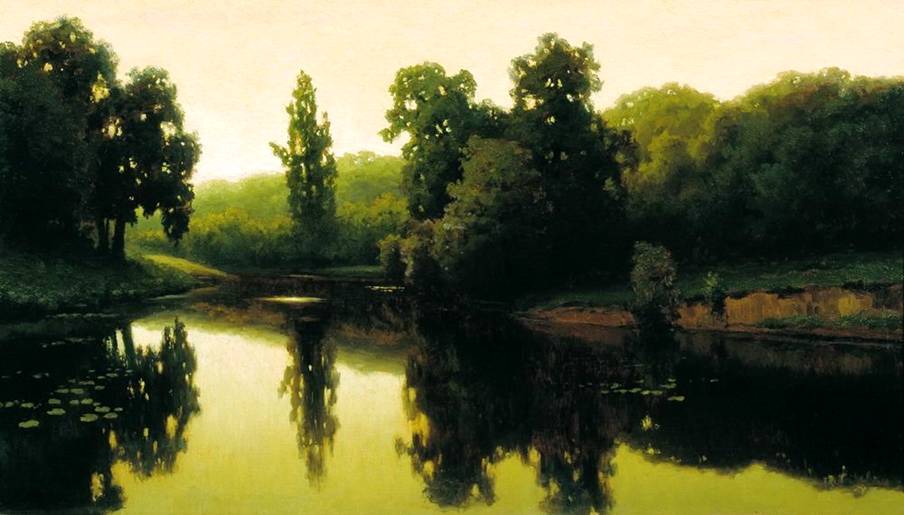The image is a highly realistic oil painting of a serene landscape scene. The dominant color palette includes various shades of green, tans, beiges, whites, browns, and blacks. At the center of the painting is a calm, almost olive-colored lake adorned with lily pads. The still water perfectly reflects the surrounding trees and the hazy beige sky, intensifying the tranquil atmosphere. To the right, a grassy cliff overlooks the lake, while more trees line the left side, adding depth to the scene. The lighting, suggestive of twilight, casts a gentle glow across the landscape, creating a unique interplay of light and shadows that highlights the lighter trees in the background. This intricate portrayal of nature, with its remarkable attention to detail in both reflection and lighting, captures the essence of a picturesque twilight moment by the lake.